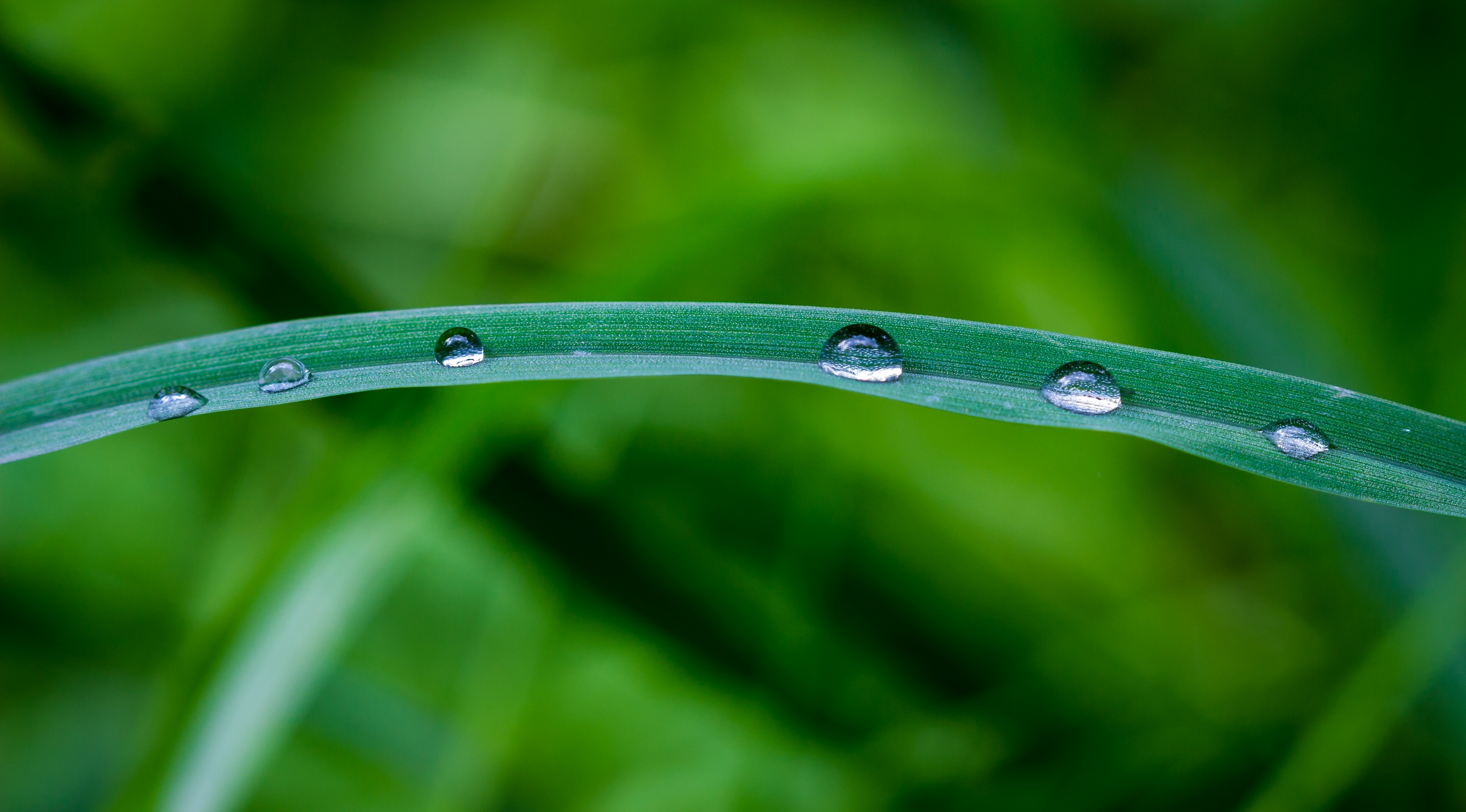This high-definition image captures a single, horizontal blade of grass extending across the center of a short and wide rectangular frame. The bluish-green blade is delicately curved, creating a natural cradle for six glistening water droplets of varying sizes, likely remnants of a recent rain shower. The background, an out-of-focus expanse, presents a lush portrayal of long, verdant grass and other slender plants, all cast in vibrant spring green hues. A darker shadowy element, perhaps from surrounding vegetation, subtly traverses the scene, enhancing the sense of an outdoor setting. The overall composition emphasizes the intricate beauty of nature, captured in exceptional detail.